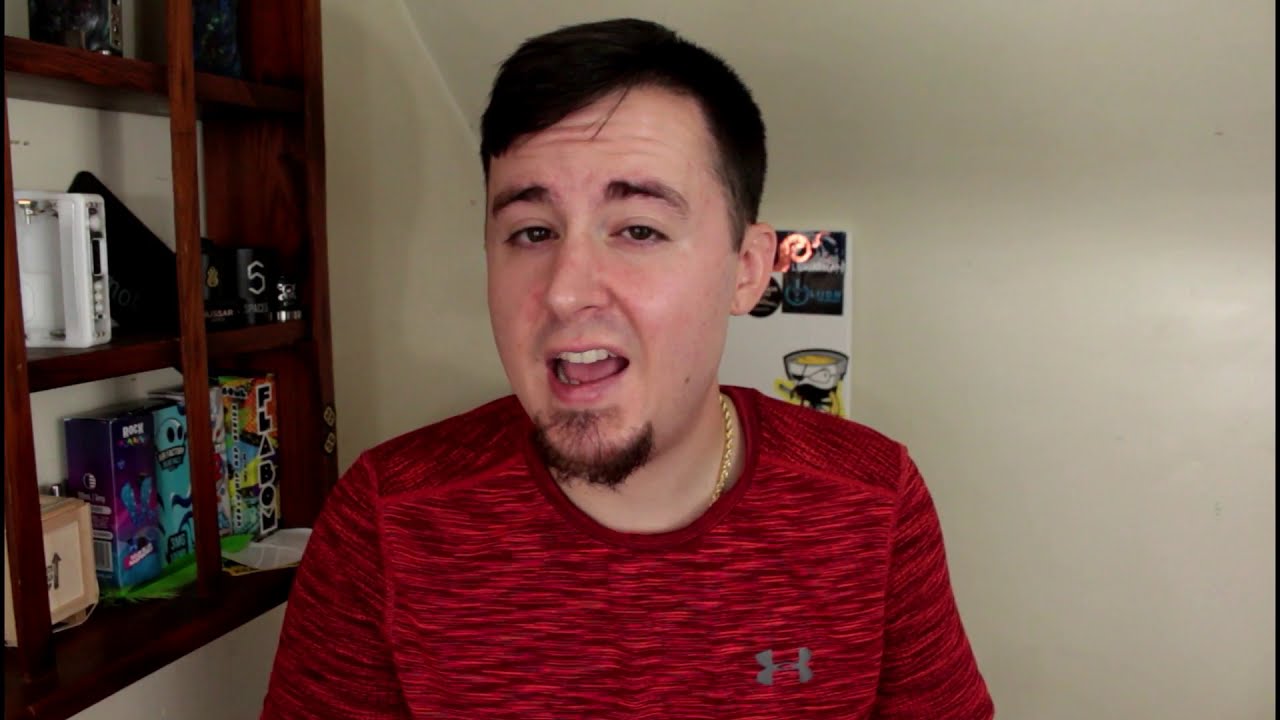This horizontal rectangular image depicts a young man, likely in his thirties, centrally positioned within a room that appears to be indoors, possibly a bedroom. He has short, dark brown hair that is slightly parted on the left, and his forehead has some horizontal wrinkles. His mouth is open, revealing his teeth and a bit of his tongue, giving the impression that he is speaking. He sports a subtle goatee and faint traces of a mustache. 

The man is dressed in a red and black heathered Under Armour t-shirt, identifiable by a grey emblem on the left side, and he wears a gold chain around his neck. Behind him, the wall is predominantly white with a poster featuring yellow, blue, and black hues. 

To his left (the image's left), a dark brown or mahogany-colored three-tiered shelf is mounted on the wall. The shelf holds various knickknacks, including a black mug marked with the number 5, a game box, and a potentially photo album-like white item on the second tier. The overall ambiance suggests a casual setting, possibly for recording or vlogging. The image's color palette includes off-white, red, black, gray, brown, white, purple, light blue, and orange.